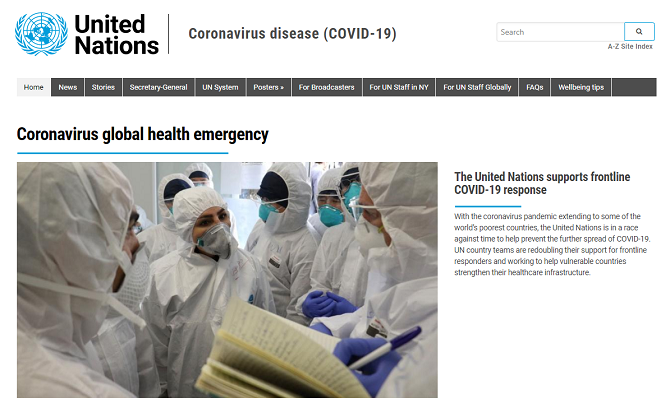The image depicts a United Nations webpage focused on the Coronavirus Disease (COVID-19). At the top of the page, the title "Corona (COVID-19)" is prominently displayed. The top right corner features a blue United Nations logo with "United Nations" written in bold black letters. 

Beneath this section is a search bar, followed by a "Disease Site Index." Below, there is a comprehensive menu bar featuring options such as Home, News Stories, Secretary General, UN System, Posters, For Broadcasters, For UN Staff in New York, For UN Staff Globally, Frequently Asked Questions, and Well-being Tips. 

In the content section, there is a headline reading "Coronavirus Global Health Emergency." Accompanying this is an image showing several people dressed in head-to-toe personal protective equipment, including masks and white suits, to guard against the virus. The foreground displays a person holding open a notebook and taking notes, seemingly engaged in a conversation with their peers. 

Next to the image, text details the United Nations' efforts to support the frontline COVID-19 response. It highlights the organization's race against time to assist some of the world's poorest countries in preventing the further spread of the virus. UN country teams are intensifying their support for frontline responders and working diligently to bolster vulnerable countries' healthcare infrastructure.